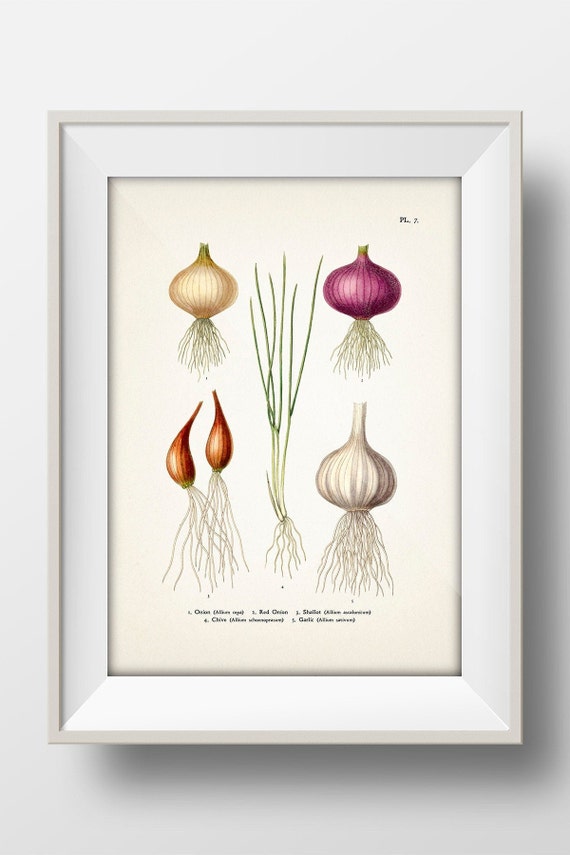The image is a detailed, color botanical artwork featuring various types of onions and garlic, framed in a white wooden frame with white matting, set against a light gray wall. The arrangement consists of four specimens: a yellow onion with a blend of yellow and white skin and visible roots at the top left; a fully intact red onion with dangling roots at the top right; a pear-shaped shallot with the point upwards and roots below at the bottom left; and a clove of garlic with multiple cloves visible and hanging roots at the bottom right. In the center, a cluster of green onions (scallions) divides the composition vertically. Each type is meticulously numbered and labeled, though the small black lettering at the bottom remains illegible. The artist's signature, "F.L.P.," is noted in the top right corner.